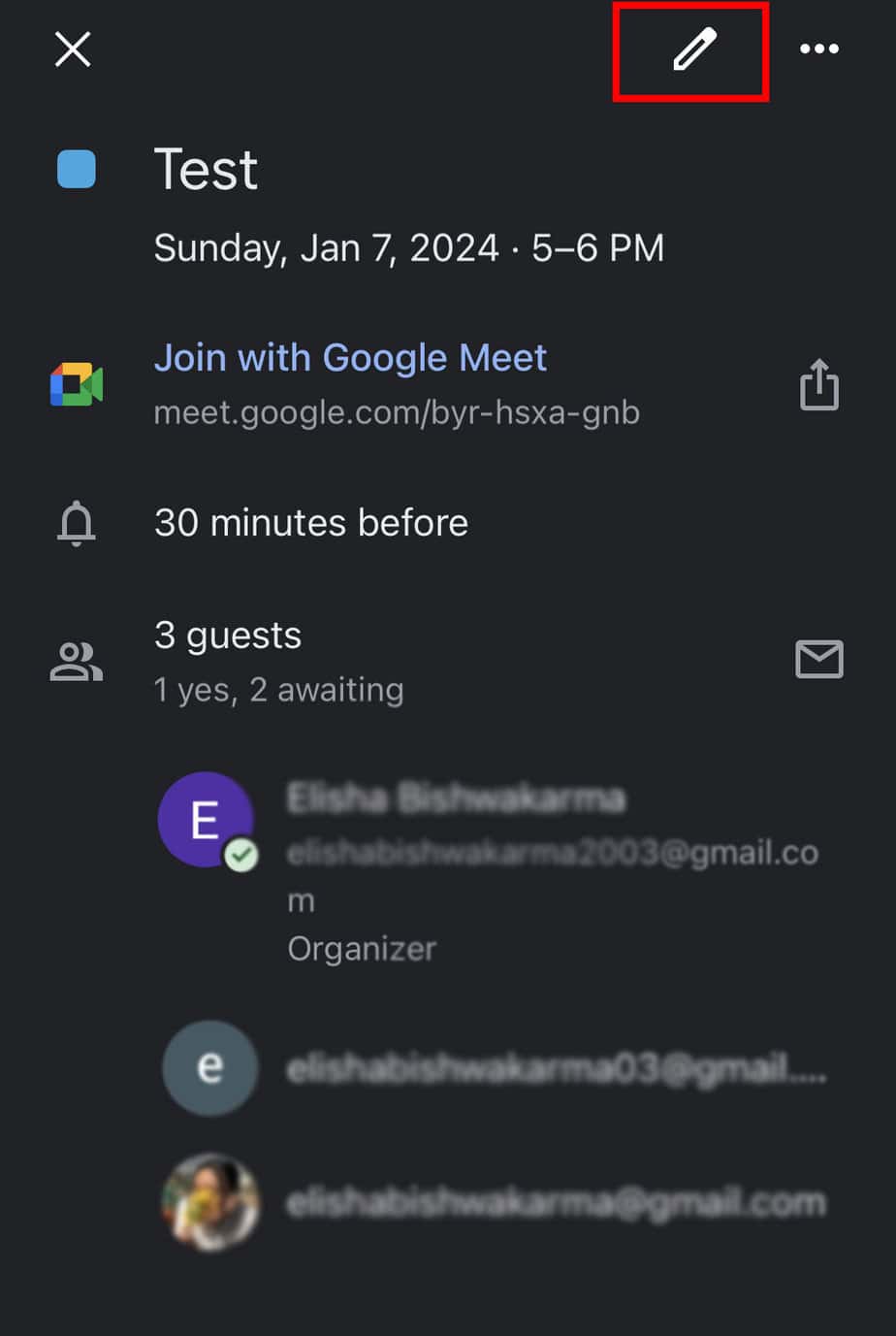The image captures a screenshot of a calendar event displayed on a smartphone. At the top, the event is labeled "Test," scheduled for Sunday, January 7th, 2024, from 5:00 to 6:00 p.m. Below the title, there's an option to join the meeting via Google Meet, highlighted in blue, with the URL "meet.google.com/BYR-HSXA-GNB." Adjacent to this link, a notification bell icon is visible, indicating a reminder set for 30 minutes before the event. Further details show a section labeled "Guests" with a status of "1 yes, 2 awaiting." There is an 'E' with a checkmark next to some guest information, which has been intentionally blurred out for privacy. The email addresses are partially visible, such as an "M" from a gmail.com address and the word "Organizer," but specific details remain obscured. Notably, an "E" within a purple circled icon and a white lowercase 'e' on a gray background are also visible. A blurred profile picture appears below these elements, ensuring the identities and email addresses of participants are kept confidential.